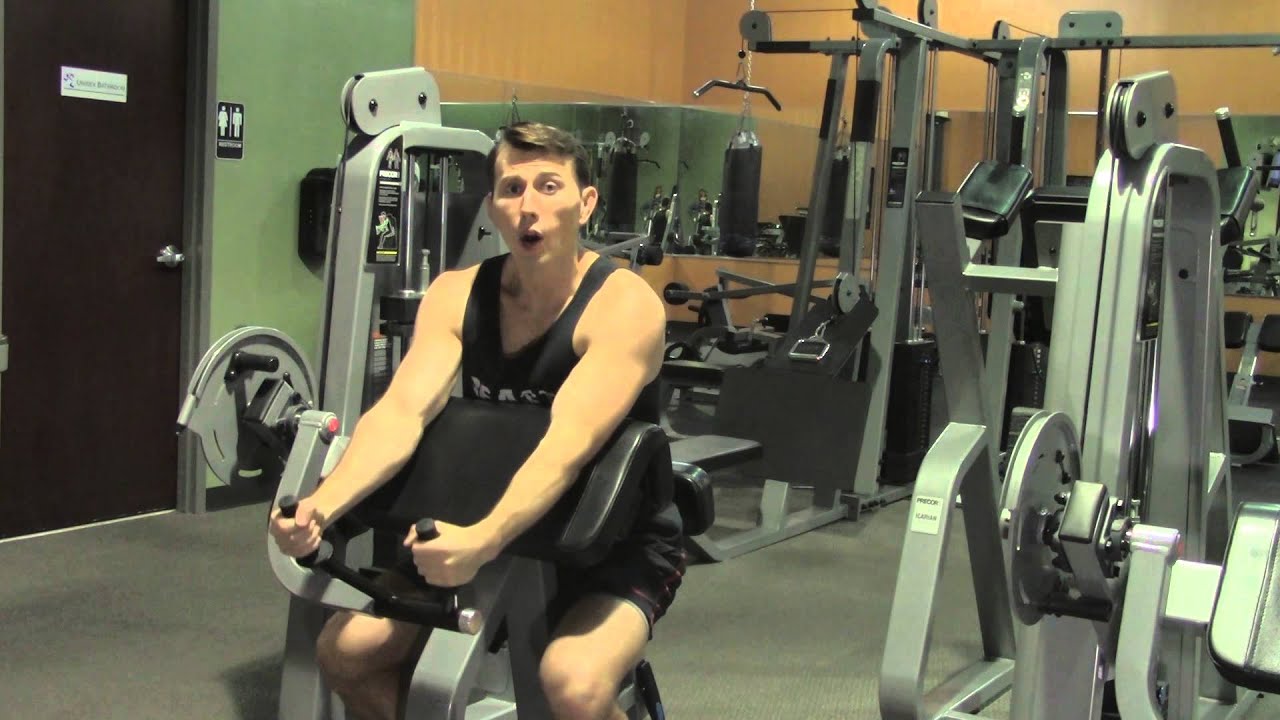The photograph captures a young man intensely working out in an unusual gym filled with robust, metal equipment. The horizontal rectangular image shows the man seated on a unique piece of exercise machinery, which he utilizes for an intense bicep workout. The machine, made of tall, green metal, resembles a bike but features just two handles and an adjustment mechanism on the side. The young man, clad in a black tank top and black shorts, has his arms extended in front of him, pushing against the machine's resistance. He gazes directly at the camera with a surprised expression, mouth slightly open. The gym's environment is striking, with an orange wall in the background, a green-teal wall adorned with mirrors that reflect other heavy metal equipment, and a brown restroom door on the left. The gym floor appears to be a gray mat, enhancing the stark, industrial feel of the space.